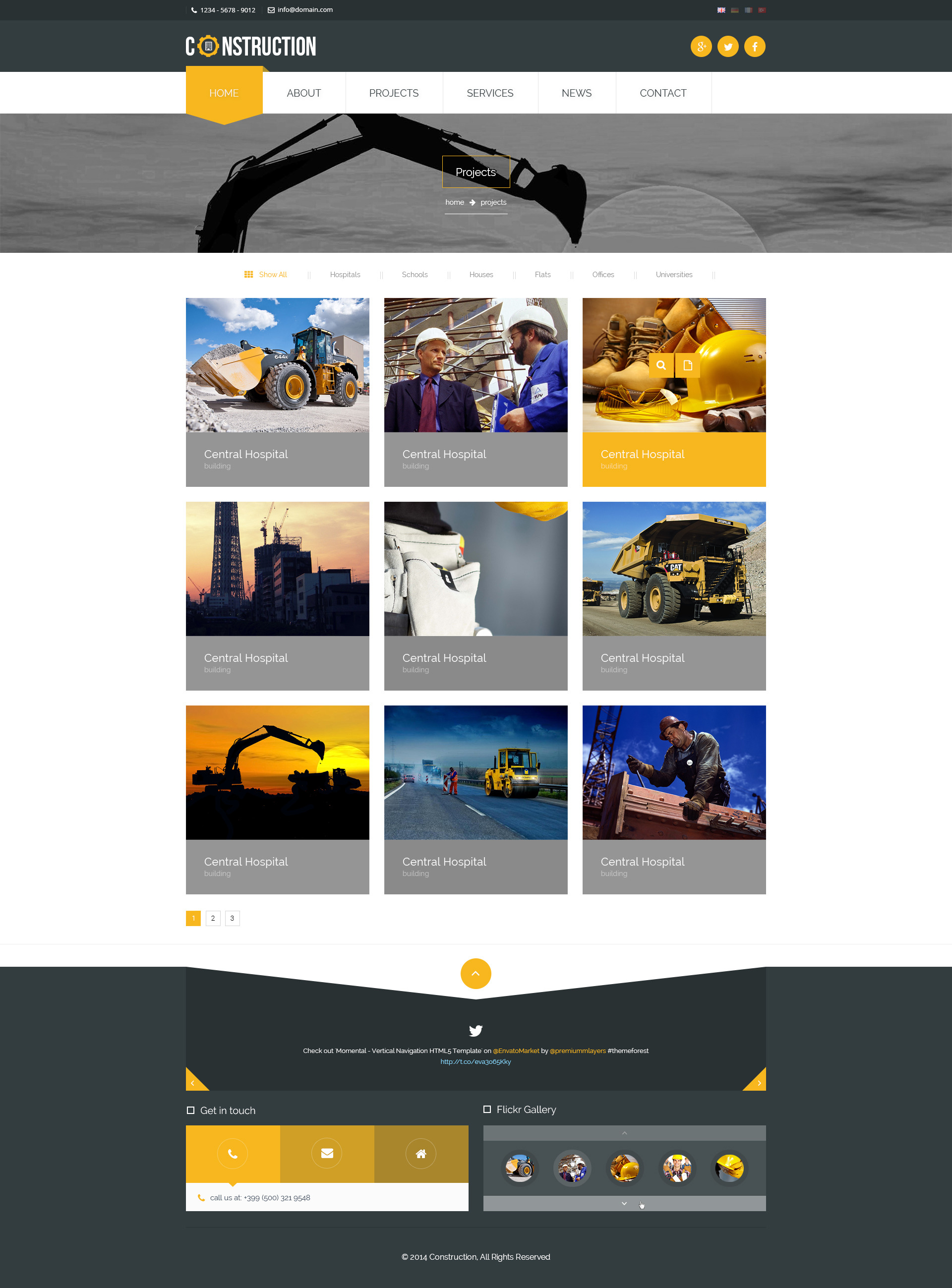**Image Description: Construction Company Website Layout**

In the top left corner of the image, the word "co-construction" is prominently displayed. The second "O" in "construction" is cleverly designed as an orange gear lever. The letters are white, placed against a black background, indicating it is the header of the webpage. 

On the top right, there are three social media icons: Google+, Twitter, and Facebook. These icons are orange while the symbols are drawn in white. Below these icons are navigational tabs to various sections of the site such as About, Projects, Services, News, and Contact. 

The active tab on the top left is "Home", which is highlighted in orange. Below "Home", there is a button labeled "Project" positioned over an image of a black excavator arm.

The main page is divided into a 3x3 grid, featuring nine distinct images:

1. **Top Left**: A yellow excavator with black tires.
2. **Top Center**: Two workers; one in a suit and one in a blue uniform, both wearing white helmets.
3. **Top Right**: A highlighted yellow helmet; this image is in full color while others are in grayscale.
4. **Center Left**: A photograph of a building.
5. **Center**: A picture of a white object.
6. **Center Right**: Another yellow excavator.
7. **Bottom Left**: An image of a black excavator silhouetted against a sunset.
8. **Bottom Center**: Yet another image featuring an excavator.
9. **Bottom Right**: A worker engaged in a task.

At the bottom of the page, there are contact options listed: "Get in touch by call, email, date". These options, along with the home button, are highlighted in orange.

This detailed layout is indicative of a structured and visually engaging website for a construction company.